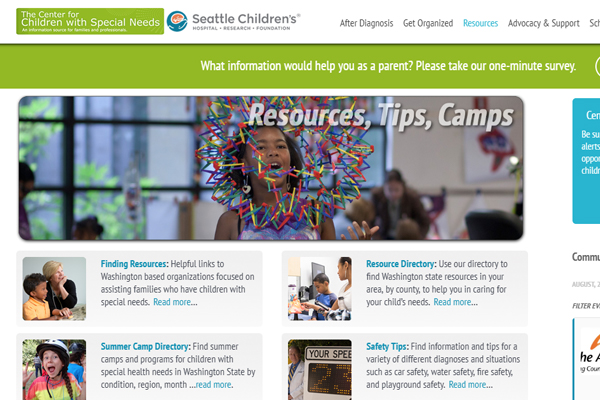The image is a low-resolution advertisement for the Center for Children with Special Needs, presented in a green box with white text at the top left. Due to the image quality, some of the smaller text is difficult to read. On the right-hand side, it displays "Seattle Children's" in gray text, followed by "Hospital, Research, and Foundation." To the left of this text, there is a blue circle encompassing a red-orange shape. 

To the right, the image reads "After Diagnosis, Get Organized" and "Resources in Blue," followed by "Advocacy and Support," all in gray text aligned horizontally. 

Below, in a green area with white text, a message prompts viewers, "What information would help you as a parent? Please take our one-minute survey." The section includes an image of a young girl gazing in amazement at a large, colorful toy forming a complex shape. This part of the image is labeled with "Resources, Tips, and Camps."

At the bottom, there are four clickable sections, each with a headline and accompanying picture of people. The sections are:
1. Top-left: "Finding Resources"
2. Top-right: "Resource Directory"
3. Bottom-left: "Summer Camp Directory"
4. Bottom-right: "Safety Tips"

Each of these sections includes a short paragraph of descriptive text.